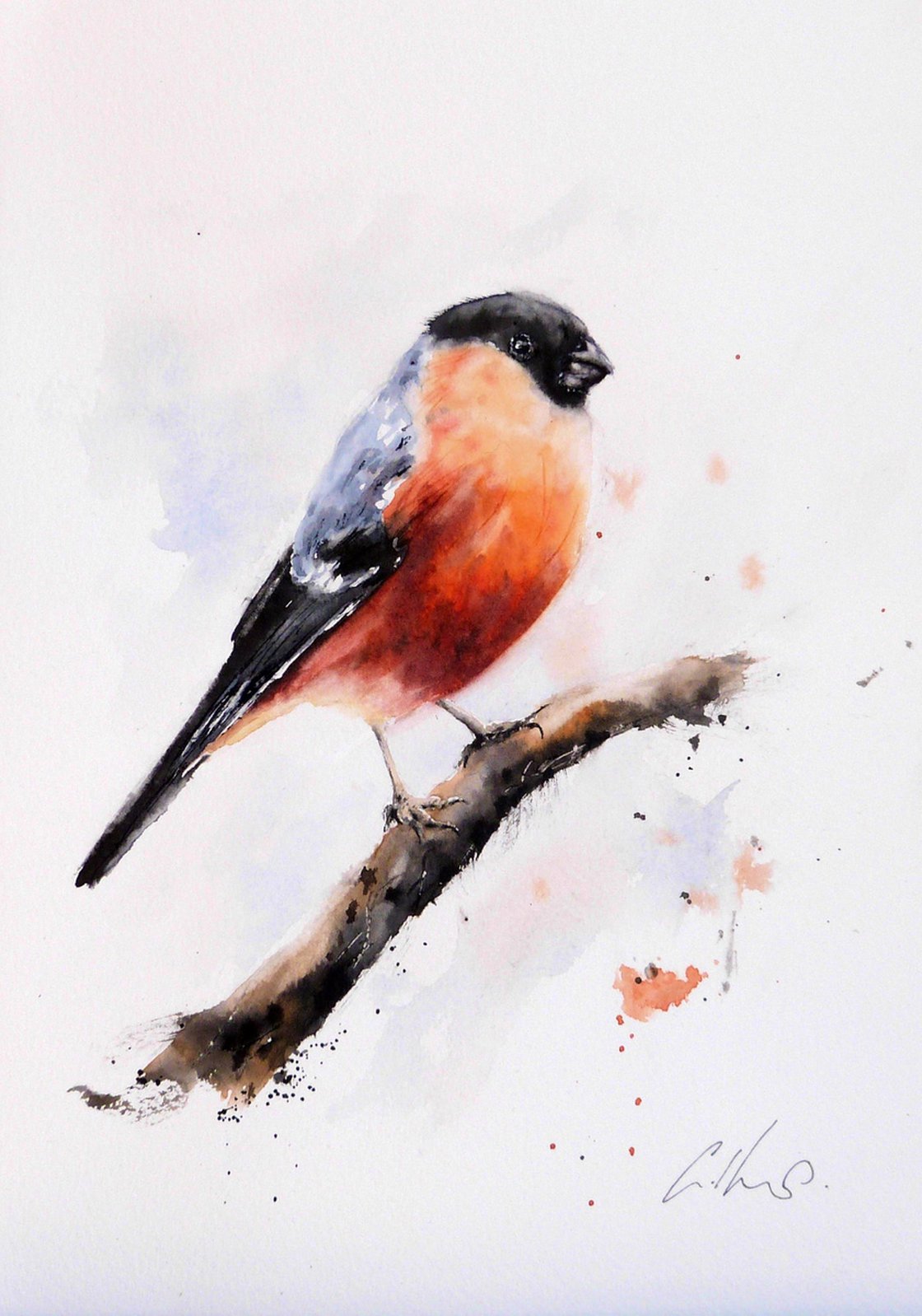The image depicts a small, plump bird, likely a robin, standing on a floating fragment of a thin tree branch. The bird's chest transitions from light orange to dark red towards the lower part, and it has a distinct black head with a shiny, reflective black eye and a short, black beak. The bird's wings are a blend of black, white, and blue, while its back also exhibits blueish tones. It has thin, yellowish legs. The background features artistic blue splotches and smudges indicative of a watercolor style, creating an impression of sky amidst an otherwise white expanse. Occasional orange and blue paint splashes are visible near the bird and the branch. The artist's signature appears in the bottom right corner, though it is somewhat difficult to decipher, resembling "C-I-H-N-S".